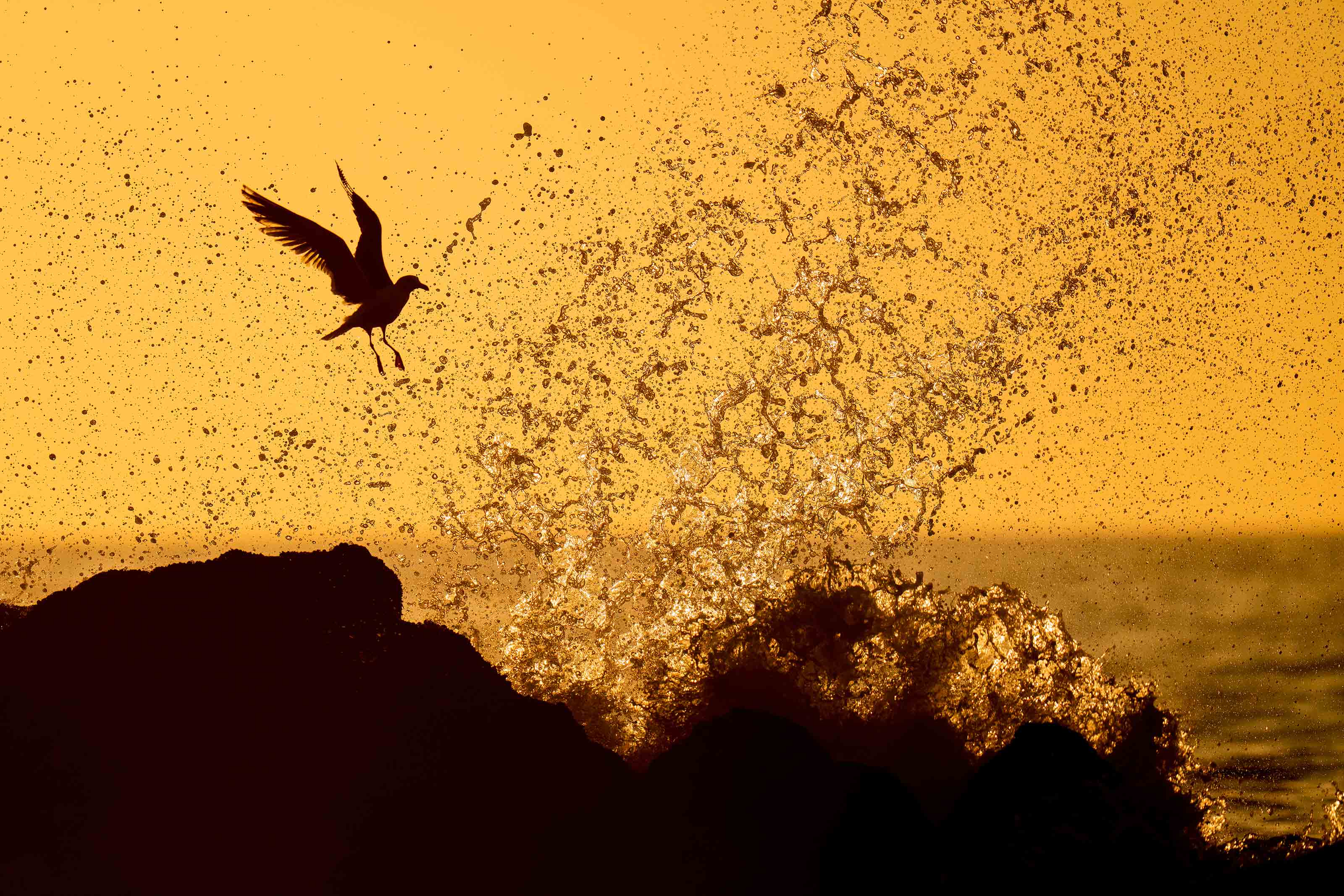This nature photograph captures a captivating scene at the beach during sunset. The sky is painted in a golden orange hue, casting a warm light over the entire scene. In the foreground, a seagull with long, pointy wings and legs flies away from the viewer, frozen in the moment with its wings stretched back as if pausing mid-flight. The dark silhouette of the bird contrasts sharply against the bright sky. Below, waves crash against a rocky shore, creating a dramatic white and dark spray of water that fans up into the air. The rocks and the bird appear as black silhouettes, adding depth to the image. The interplay of dark and light gives the scene a sense of motion and tranquility, while the background showcases the shimmering water with grey and yellowish tones. The only colors visible in the image are shades of golden orange, brown, black, and bursts of white from the crashing waves, emphasizing the scenic beauty of the seaside sunset.